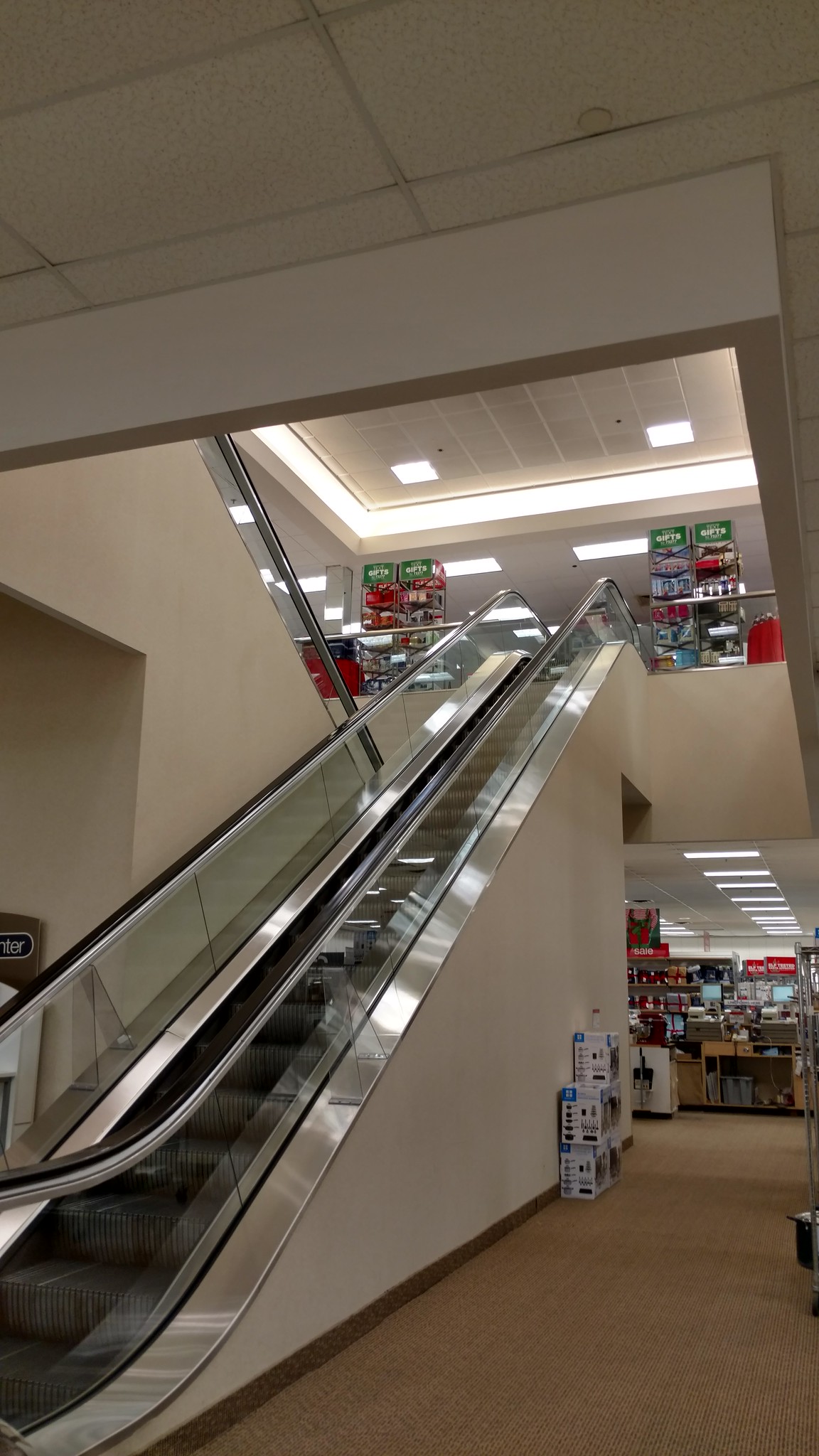The image depicts the interior of a two-story retail store, captured within a vertically rectangular frame. The photograph is taken from the first floor. On the lower right side, a narrow path covered in brown carpeting leads the viewer’s eye through the scene. Dominating the composition, an escalator stretches diagonally from the bottom left corner to the center right, inviting customers to the upper-level shopping area. In the upper right section of the image, product display shelves are neatly arranged, showcasing an assortment of merchandise under the bright ceiling lights. The ceiling itself is a light, neutral color, complementing the overall warm and inviting ambiance of the store.